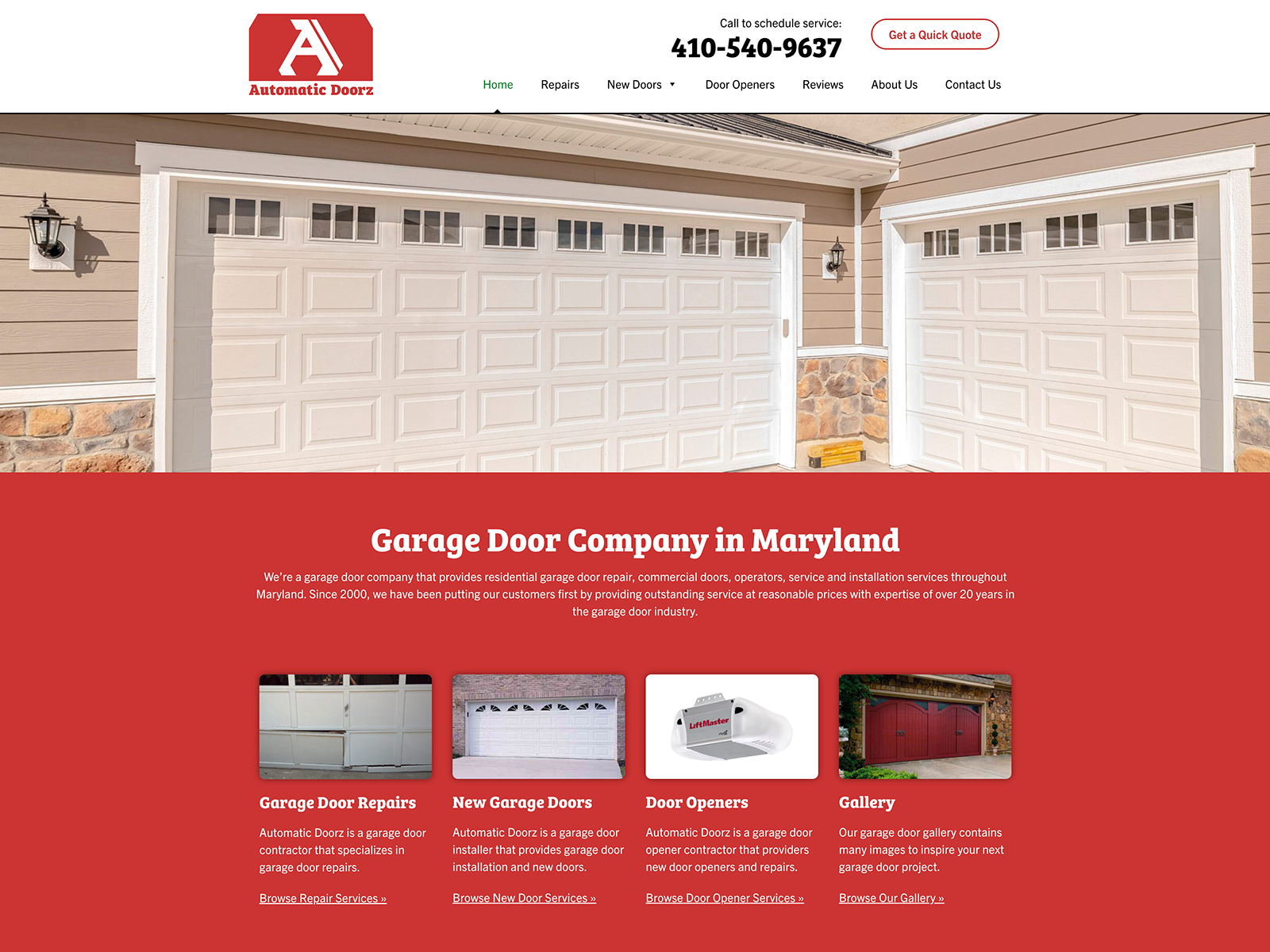The image is a screenshot from the website of the Automatic Doors Company, prominently featuring its layout and branding. In the upper left-hand corner, the company's name, "Automatic Doors," is displayed in red font within the top bar, accompanied by their logo – a stylized "A" set within a red, house-shaped box. Directly below this logo and name is the horizontal navigation menu, which includes the options: Home, Repairs, New Doors, Door Openers, Reviews, About Us, and Contact Us.

To the right of the navigation menu, there is a call-to-action message reading "Call to Schedule Services: 410-540-9637" and a "Get a Quick Quote" button. Below this, the Home option is highlighted in the menu, indicating the current page that's open. The main content area features an image of two garage doors: one directly facing the camera, and the other oriented towards the left, positioned on the right side of the image.